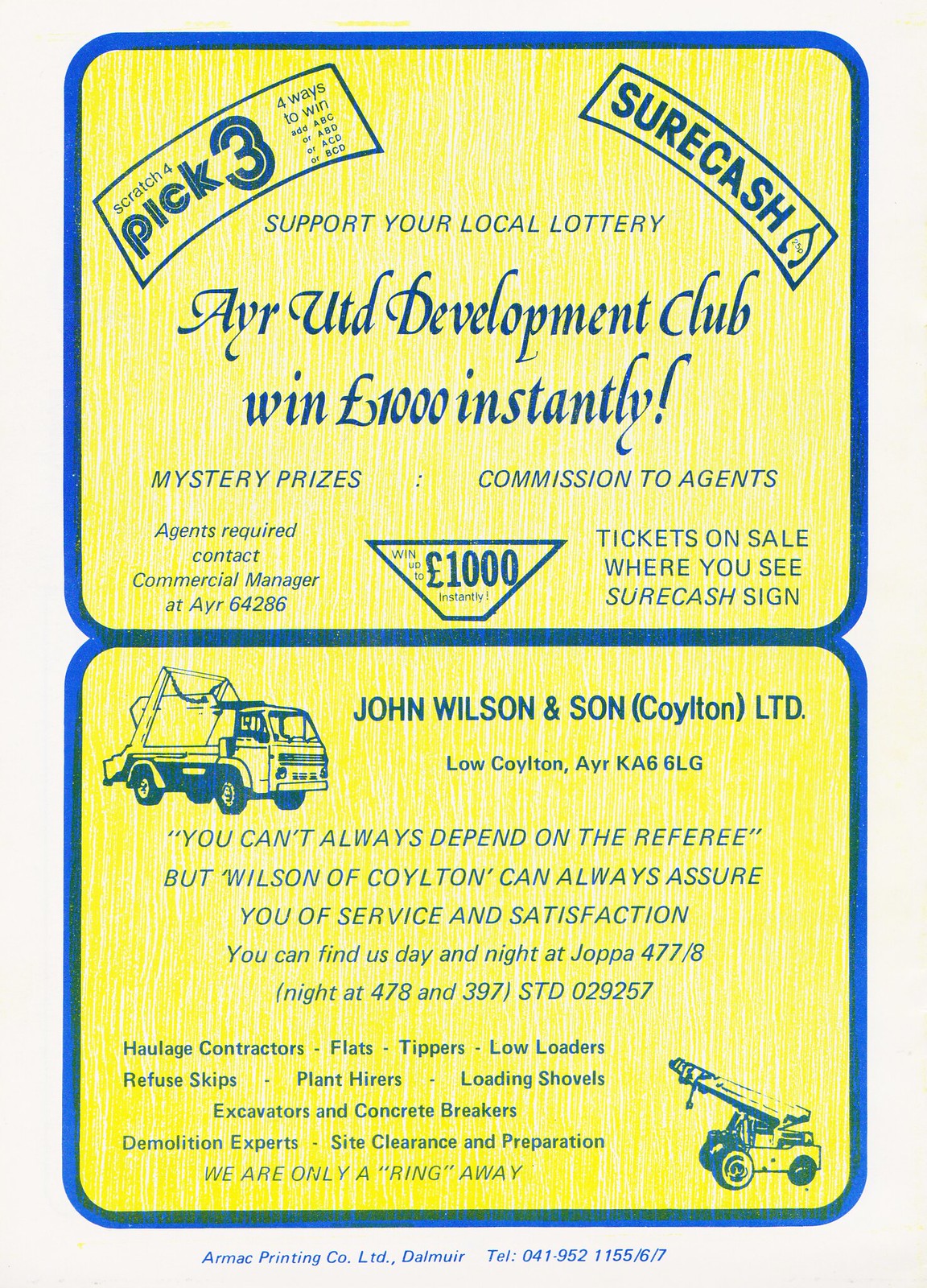The advertisement page features two prominent ads stacked vertically, set against a light gray border that frames the entire image. Each ad is positioned within a yellow rectangle bordered in blue. The top yellow rectangle promotes the AYR UTD Development Club lottery. It includes blue text with various enticing details: "Support your local lottery," "Win £1,000 instantly," "Mystery prizes," and "Commission to agents." The ad also emphasizes that agents are required and provides a contact, "Commercial Manager at AYR 64286." The lottery offers multiple chances to win with phrases like "Scratch four, pick three," and tickets available where Sure Cash signs are visible.

The ad positioned below is for John Wilson and Son, Quailton Limited, located in Low Quailton. It features the tagline, "You can't always depend on the referee, but Wilson of Quailton can always assure you of service and satisfaction." It highlights the company's extensive services, including haulage contracting, flatbeds, tippers, low loaders, refuse skips, plant hires, loading shovels, excavators, concrete breakers, demolition services, and site clearing and preparation. Contact information includes Joppa 477-8 day and night contactable at 478 and 397, with the STD code 029257.

At the very bottom of the page and within the light gray border is blue text that reads, "RMAC Printing Co., Ltd., Dalmyer, Tel, 041-952-1155-6-7," indicating the printing company responsible for the advertisement.